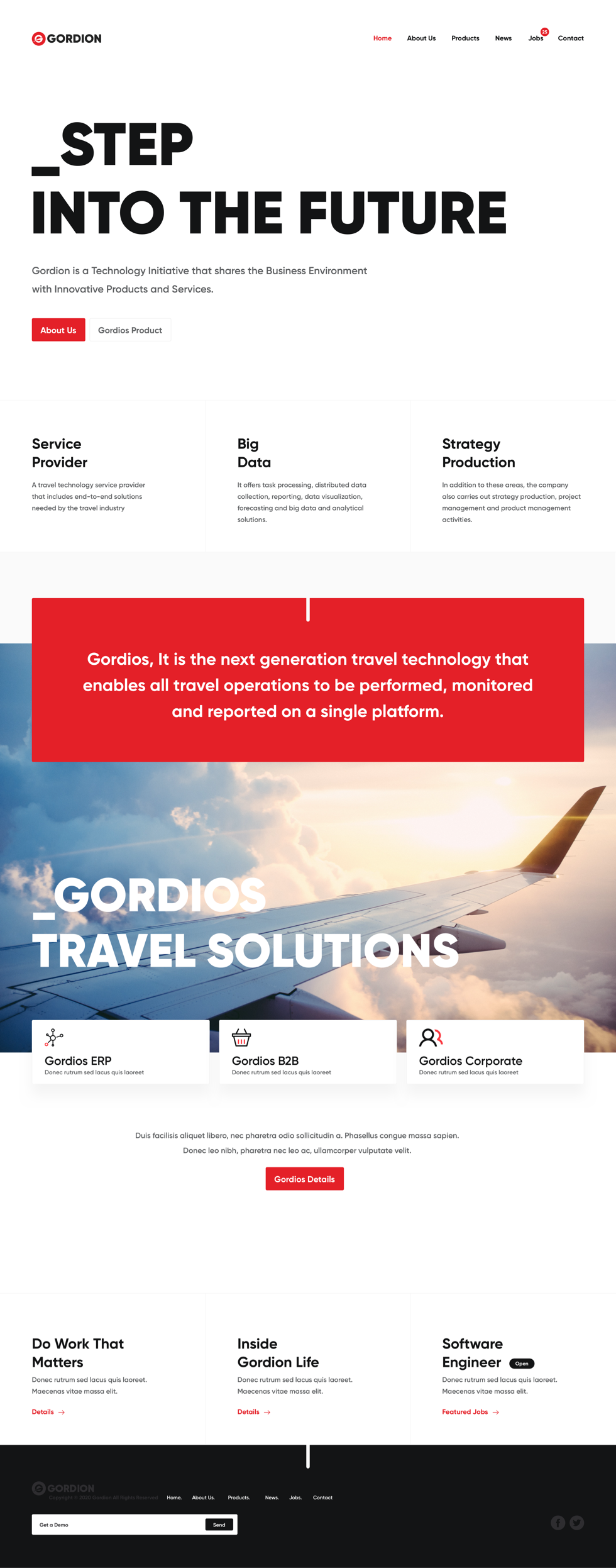Top left corner features a prominent red logo labeled "Gordian". The website navigation bar includes sections such as Home, About Us, Products, News, Jobs, and Contact. Emphasizing a forward-thinking approach, the main banner reads: "Stepping into the Future - Forward Line." This reflects Gordian's commitment to revolutionizing the business environment with cutting-edge products and services.

A striking red rectangle highlights the "About Us" section, while a white rectangle marks "Gordo's Products". Gordian is a service provider specializing in travel technology, offering comprehensive end-to-end solutions tailored to the travel industry. Their services encompass task processing, distributed data collection, reporting, data visualization, forecasting, big data analytical solutions, strategy, and production.

Additionally, Gordian excels in project management and prior management activities. The tagline "Gordo's is the next generation travel technology that enables all travel options to be formed on an impressive platform" underscores the innovative nature of their solutions. 

Highlighted travel solutions under the branding "Gordo's" include ERP, B2B, and corporate services, presented against a backdrop of an airplane wing beneath a clear sky, symbolizing innovation and boundless possibilities. The caption concludes with an inspiring call to action for prospective employees: "Do work that matters inside Gordo's - Software Engineer."

Navigation reminder: Home, About Us, Products, News, Jobs, Contact.